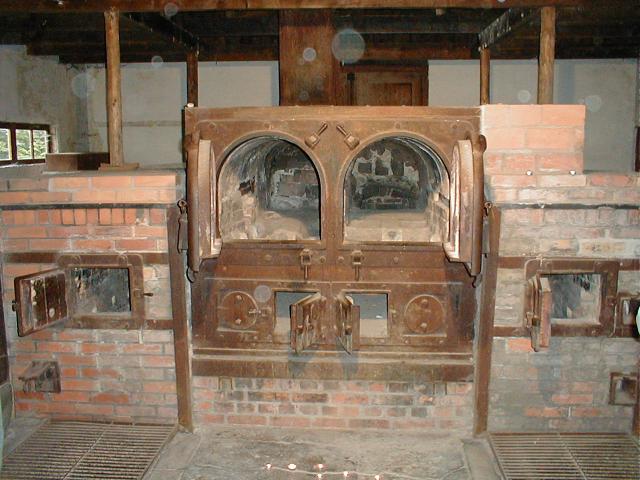The photograph captures a rustic, old-fashioned oven setup, characterized by four brick-lined ovens set into a weathered, dusty, and sooty structure. At the center, two large arch-shaped ovens with dark brown curved metal doors showcase an interior streaked with gray and beige, likely from oxidation and soot buildup over time. Below these arches, two smaller doors, presumably for feeding firewood, share the same aged aesthetic. On either side of this central piece, two smaller square ovens with brick facades, one notably more gray due to accumulated grime, are visible, each featuring soot-covered metal grates. The entire setup is supported by brickwork and wood or metal beams, with additional support poles visible in the background. The white brick-lined walls and a small window on the left, revealing green foliage and sunlight, enhance the scene's timeless, museum-like ambiance. Above, dark brown wood beams run across the ceiling, completing the picture of an antiquated, yet carefully preserved culinary apparatus.